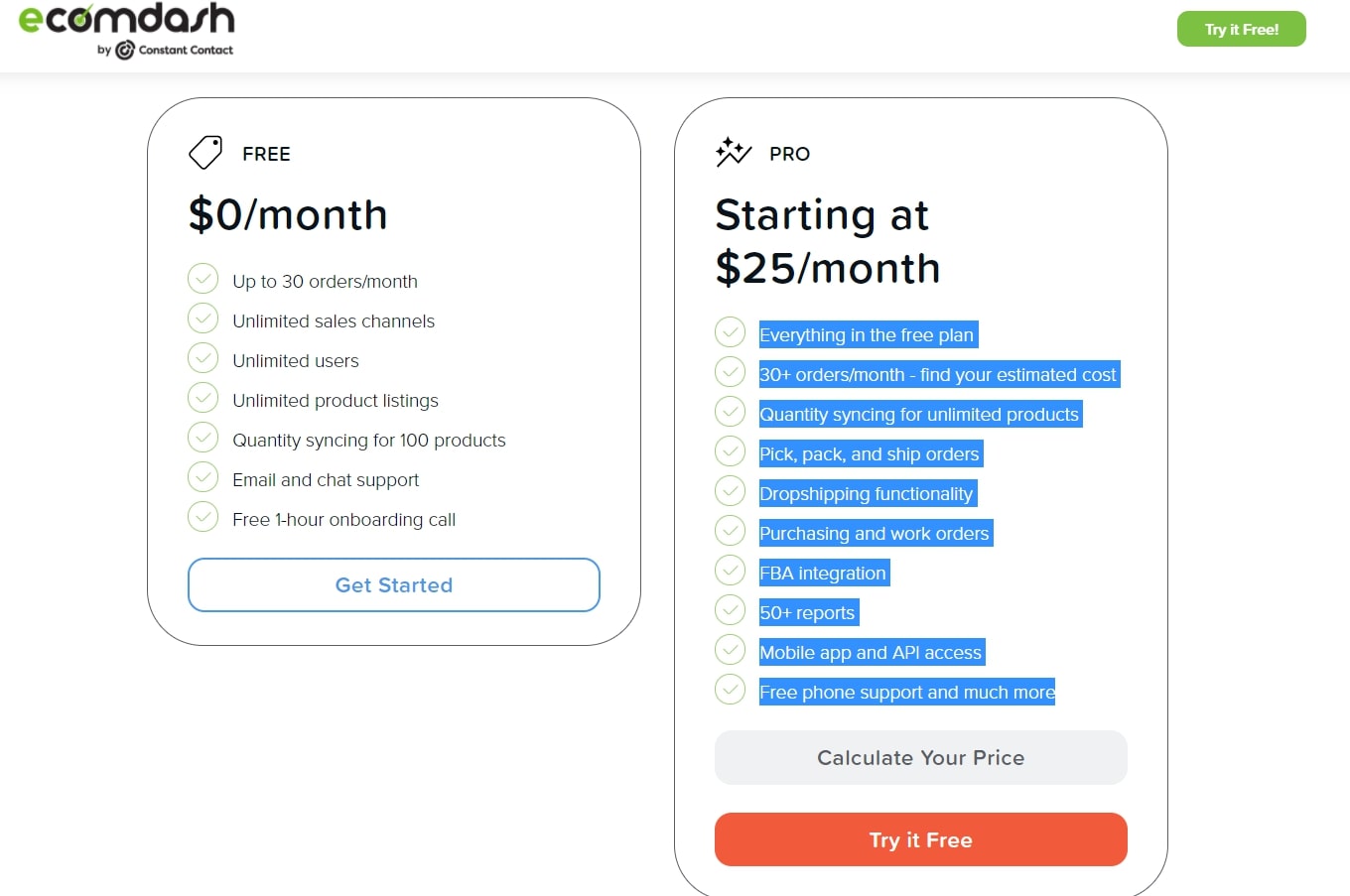This image is a screen capture from Ecomdash, a platform by Constant Contact, showcasing different types of subscription plans. The top left corner of the image features the Ecomdash logo, while the top right has a prominent green "Try It Free" button. 

The plans are as follows:

1. **Free Plan**:
   - Pricing: $0 per month
   - Features:
     - Up to 30 orders per month
     - Unlimited sales channels
     - Unlimited users
     - Unlimited product listings
     - Quantity syncing for 100 products
     - Email and chat support
     - Free one-hour onboarding call
     
   Users are encouraged to "Get Started" with this plan.

2. **Pro Plan**:
   - Pricing: Starting at $25 per month
   - Includes all features from the Free Plan, plus:
     - Over 30 orders per month
     - Quantity syncing for unlimited products
     - Pick, pack, and ship orders
     - Dropshipping functionality
     - Purchasing and work orders
     - FBA (Fulfillment by Amazon) integration
     - Access to over 50 reports
     - Mobile app and API access
     - Free phone support and more

   There is a gray "Calculate Your Price" button under this plan, and a red "Try It Free" button beneath that.

The detailed layout and color-coded buttons provide clear options for users to choose the subscription plan that best fits their needs.